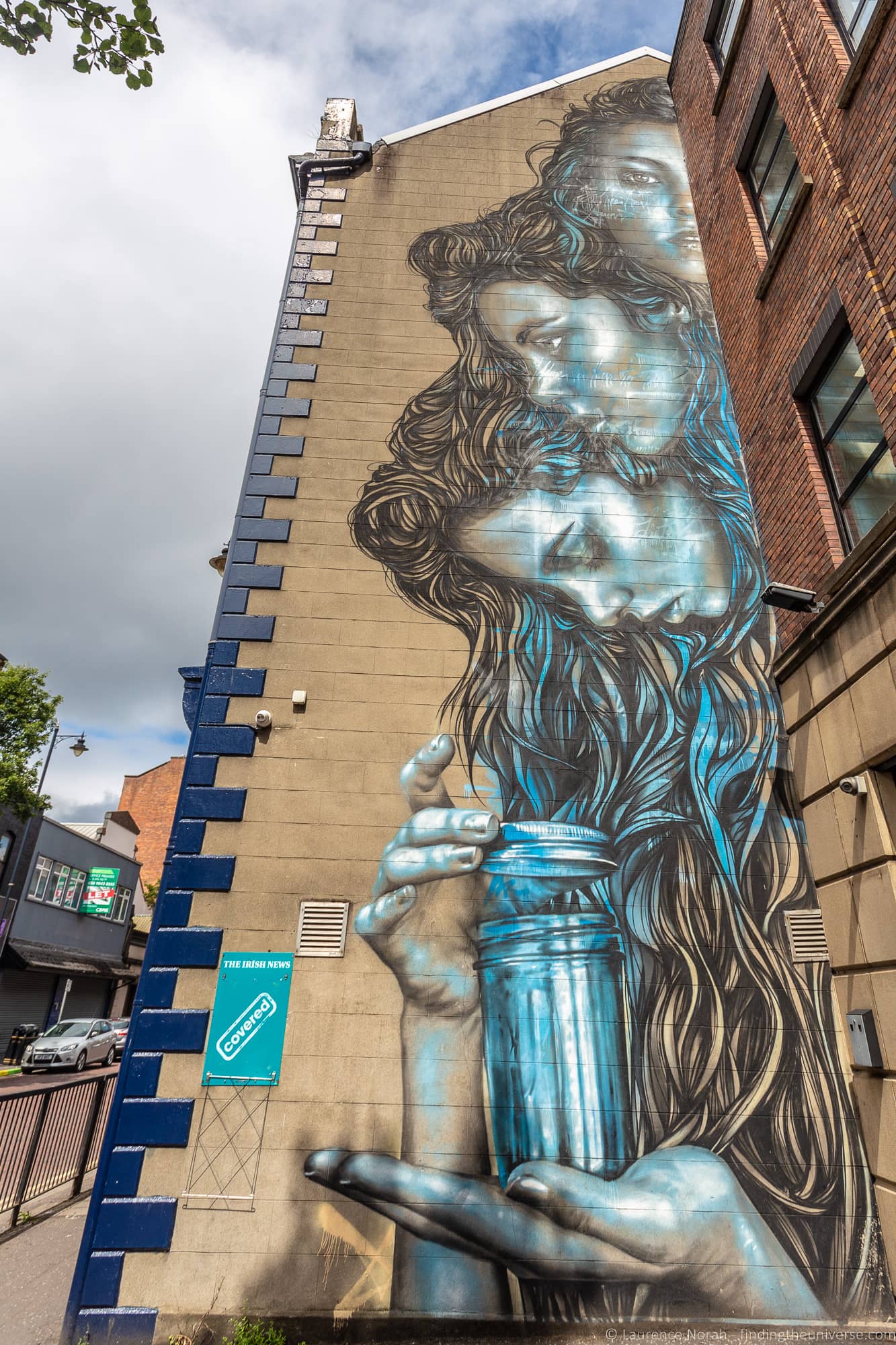The image showcases a captivating mural on the side of a multi-story, tan brick building with a distinctive blue brick border on the left side. The mural, spanning the height of the building, features three faces of women with flowing, curly hair accentuated by black lines and vibrant blue highlights. Starting from the top, the first woman’s face, positioned just beneath the rooftop point, shows only the right half, framed by medium-length curly hair. Below her, another woman is depicted with her head bent down and facing left; only the left side of her face is visible, with brown curly hair cascading down. Beneath her is a third woman, also gazing downward, showcasing a mix of light-colored hair with striking blue streaks. Her hair extends to the bottom of the building. 

In front of this last figure, a hand emerges from the building's bottom right, holding a tin canister with a silver lid slightly removed. The mural boasts an airbrushed look that makes the skin of the figures appear to radiate.

The setting is outdoors, bathed in daylight, showing a lively street scene to the left with several buildings, parked cars, and signs suggesting commercial establishments, possibly a bar. A reddish brick building on the right partially obstructs the view of the mural, enhancing the scene's urban depth. The top of the mural-building features a white vinyl roof trim that accentuates its pointed roofline, contributing to the artistic and architectural interest of the image.